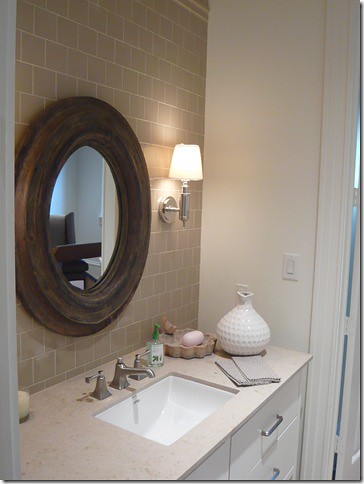A well-appointed bathroom features a pristine white sink and vanity set against crisp white walls. The vanity is equipped with white cabinets adorned with sleek silver pull handles. The central white sink boasts a brushed nickel faucet and matching handles on either side. Adding a touch of warmth, the beige countertop complements the surrounding decor seamlessly. Above the countertop, a backsplash of subway tiles in a light brown and white mosaic pattern enhances the aesthetic, creating a harmonious blend with the walls and vanity top.

A round, brown, oval-shaped mirror is positioned directly above the sink, reflecting the room's stylish elements. A mounted light fixture on the tiled wall next to the mirror provides ample illumination. The vanity top is tastefully decorated with a selection of items: a white vase, fancy napkins, a small dish, and a clear soap dispenser placed to the right of the faucet. The soft glow of the light fixture highlights these details, while a light switch is visible on the adjacent wall. An open door in the background allows a glimpse of natural light streaming in, adding a subtle touch of brightness to the predominantly beige, brown, and white color scheme.